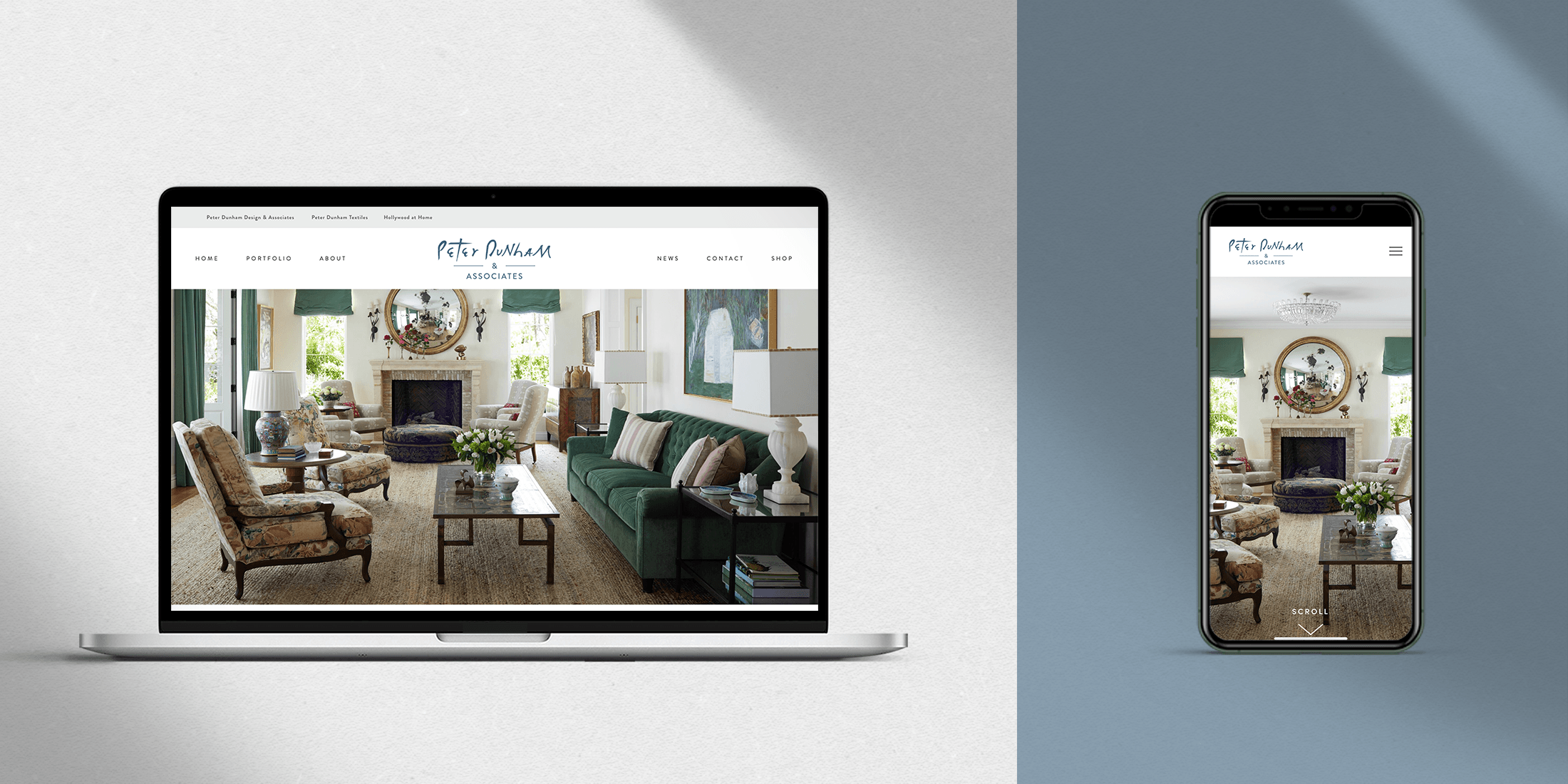This photo showcases a laptop positioned on the left against a gray background. The laptop screen features a detailed image of a living room furnished with a green couch, green blinds over the windows, and a white-walled interior. Dominating the back wall is a large round mirror hanging above a fireplace. The room is lit by lamps with white-colored lampshades; one lamp, situated on a table to the left, has a green base. Two brown cushioned chairs flank a central brown wooden table adorned with green leaves, white flowers, and various pieces of glassware. A table to the right is topped with a stack of books. All of this rests on a brown floor.

The laptop is sleek, with a black border around the screen and a silver base. Adjacent to the laptop, on the right, is a phone set against a greenish blue-gray background. The phone screen displays a shrunken version of the same living room image, where only parts of the chairs are visible and the couch is out of view. At the bottom of the phone screen, an arrow accompanies the word "scroll." Both screens prominently feature the website "Peter Dunham and Associates," along with menu options: Home, Portfolio, About, News, Contact, and Shop.